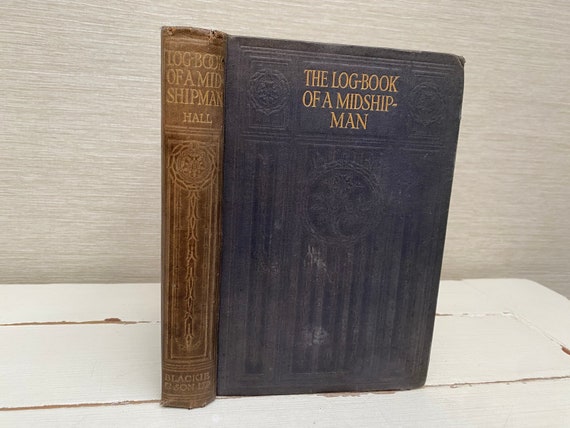The image depicts a rectangular, antique book, with a prominent cover and spine. The title, "The Log Book of a Midshipman" by Hall, is embossed in gold lettering on a textured black background. Elegant, elongated lines and intricate designs adorn the front cover, capturing the eye with a sense of historical craftsmanship. The spine of the book, also detailed in gold, echoes the title and author's name, reinforcing its venerable appearance. The book is positioned on a pristine, bright white shelf, against a soft tan backdrop reminiscent of aged vanilla. The overall aesthetic suggests this tome is an artifact from the shipping industry, perhaps dating back two centuries, embodying the maritime legacy it chronicles.